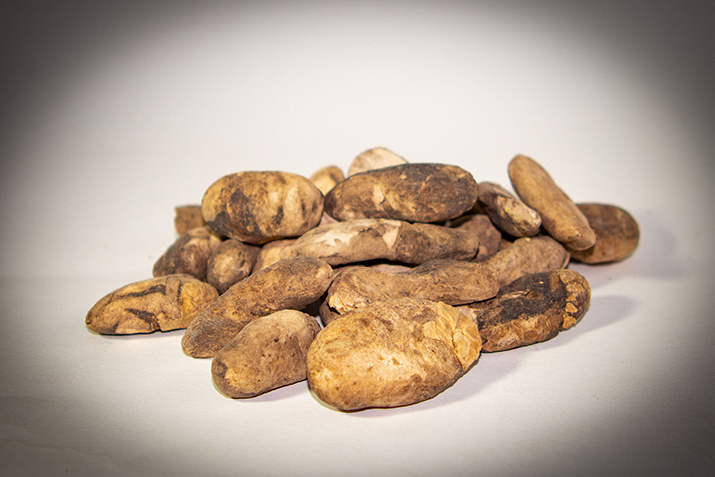The image features a substantial pile of at least 30 potatoes, stacked haphazardly on a white surface, illuminated dramatically as if by a spotlight. The potatoes vary in shape and size, with some appearing flat and others more traditionally oval. Their color palette spans a range of browns, from light golden hues to darker, almost dirty-looking shades. The foreground potato stands out with a golden brown tint, while those towards the back are darker. The photograph has a subtle vignette effect, with dark gray corners fading into the image, drawing the viewer's attention to the textured and varied pile of potatoes.